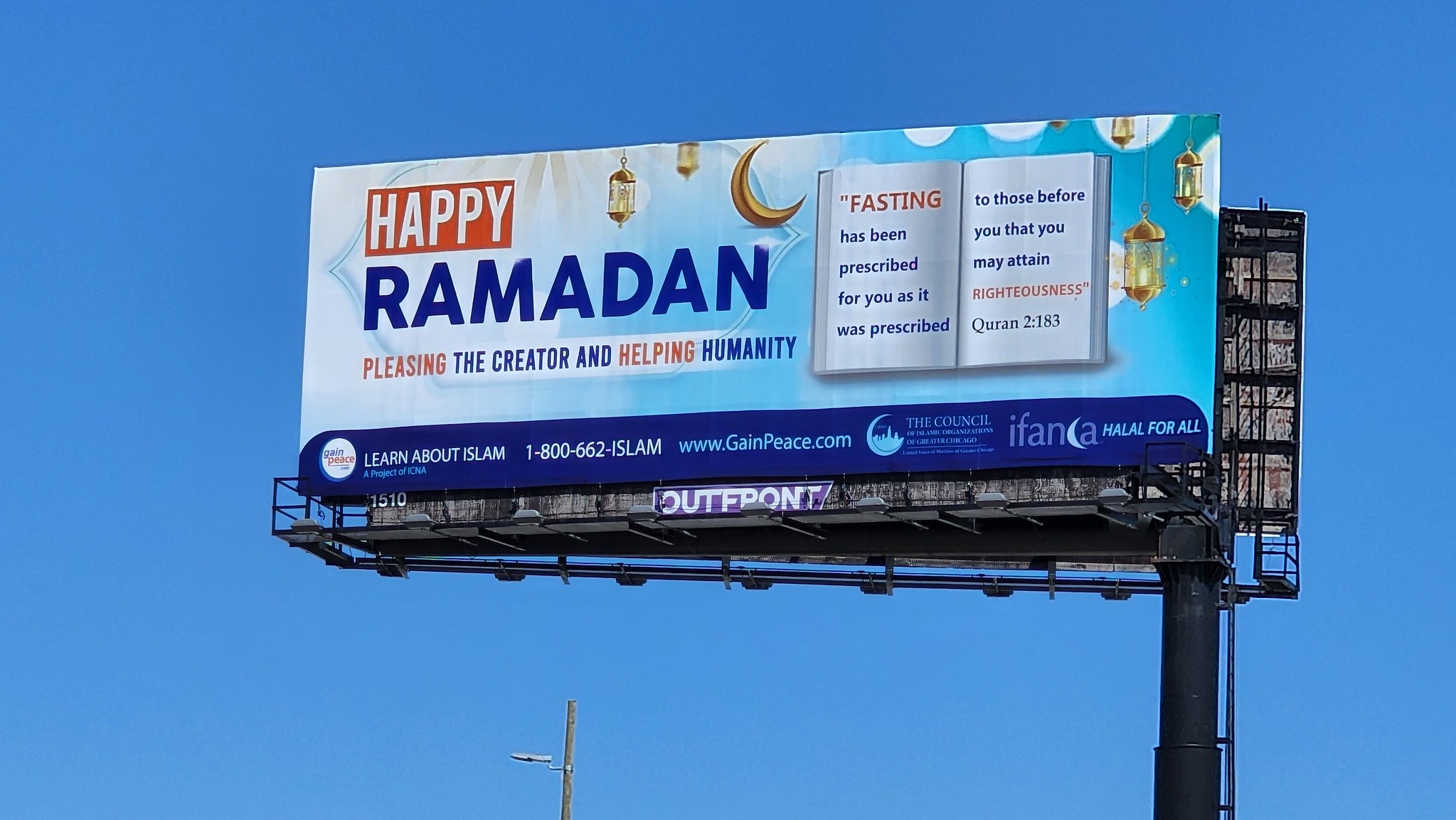A vibrant photograph captures an urban skyline dominated by a prominently placed billboard at the forefront. This billboard stands atop a sturdy, black metal post which leads to a walkway on one side. The billboard itself features a harmonious combination of colors and messages; a striking purple section displays the phrase "Out Front," while the central area, adorned in serene blue and white hues, reads, "Happy Ramadan," alongside the encouraging words, "Pleasing the creator and helping humanity. Fasting has been prescribed for you as it was prescribed to those before you, that you may attain righteousness. - Quran 2:183." The visual appeal is enhanced by decorative elements including a delicate crescent shape and elegant golden lanterns, imparting a sense of celebration and reverence. Contact information is provided beneath, inviting onlookers to learn more about Islam at "1-800-662-ISLAM" or by visiting "www.gamepeace.com." In the background, under a clear, cloudless blue sky, the top of a brown power line can be seen, equipped with a streetlight, adding an element of urban infrastructure to the peaceful scene.